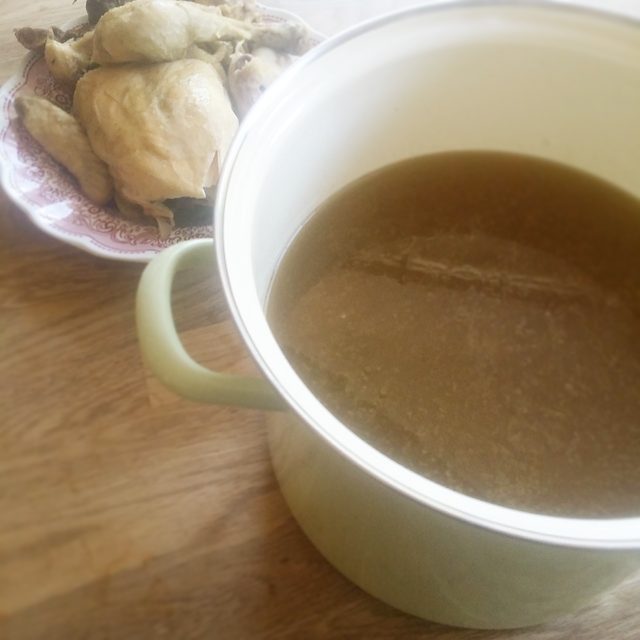In a hazy, slightly foggy photo that appears to be taken in a kitchen, we see a light green tall stock pot with a white interior, filled about halfway with an opaque brown liquid, possibly gravy. This stock pot sits on a brown wood grain table. Behind it, there's a white plate adorned with a dark red, wavy design. The plate is piled high with dismembered cooked chicken parts, including the breast, wings, and a leg resting on top. The chicken appears a bit dry, suggesting it may have been soaking in the pot's liquid. The scene captures a moment in someone's home, showcasing a freshly made meal possibly intended to feature chicken and gravy.